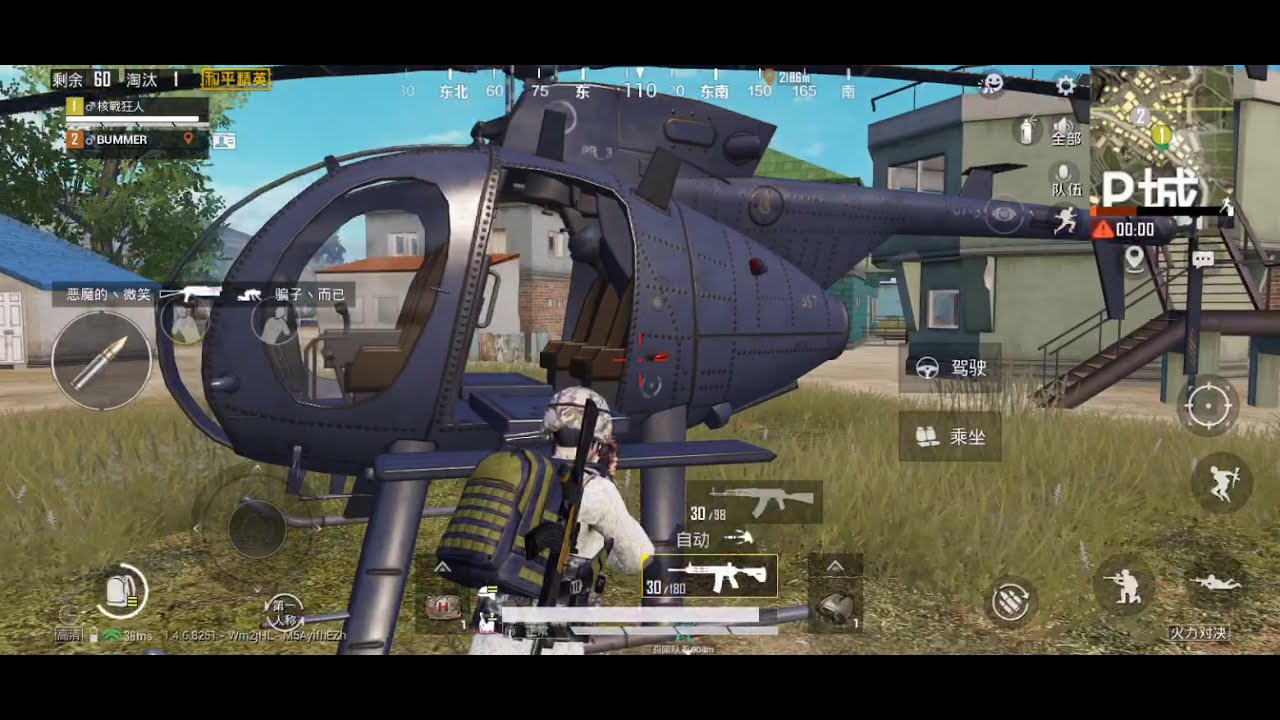The image is a detailed screenshot of a mobile shooter video game, evident from the on-screen controls and commands, which appear to be in Chinese. Central to the scene is a dark blue-gray helicopter with riveted metal plates, sitting broadside with its tail pointing to the right. Next to the helicopter stands a player character, clad in a white military uniform, army helmet, and a large green backpack with black outlines. The character has a rifle slung over their shoulder and might be holding binoculars or another object. The helicopter is positioned on a grassy area, and behind it, buildings are visible, with metal stairs leading to different platforms on the right. Overlaying the image are various game icons, including a white gun icon in a translucent gray rectangle near the character. In the upper left corner of the screen, nicknames of players are displayed, one in Chinese and another named Billmer.